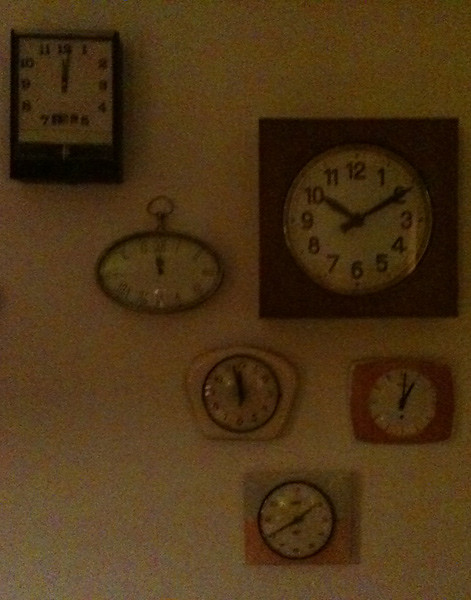This grainy, dimly lit colour photograph captures six distinct clocks on a beige wall with red flecks. The uneven lighting makes the wall appear grainy, as though the picture was taken at night in poor lighting. Each clock has a unique design and is scattered across the wall without a consistent pattern, but their spacing is relatively even. 

In the upper left corner, there is a square clock with hands pointing to 12:00. Just below it and slightly to the right, an oval clock also shows the time as 12:00. Directly to the right of this oval clock is a square-framed clock with a circular white clock face, set to 10:10. Below this, off-centre on the wall, is a clock resembling a slice of bread in shape but circular in the middle, its hands pointing to almost 12:00. Adjacent to this on the right edge is a reddish square clock with a round clock face, showing the time as 1:00. Finally, at the bottom right of the arrangement, there is another square clock with a grey and orangey-red frame; the round white clock face inside displays 1:40.

Despite the varied shapes and styles of the clocks, they create a visually intriguing yet disorderly display on the textured wall.